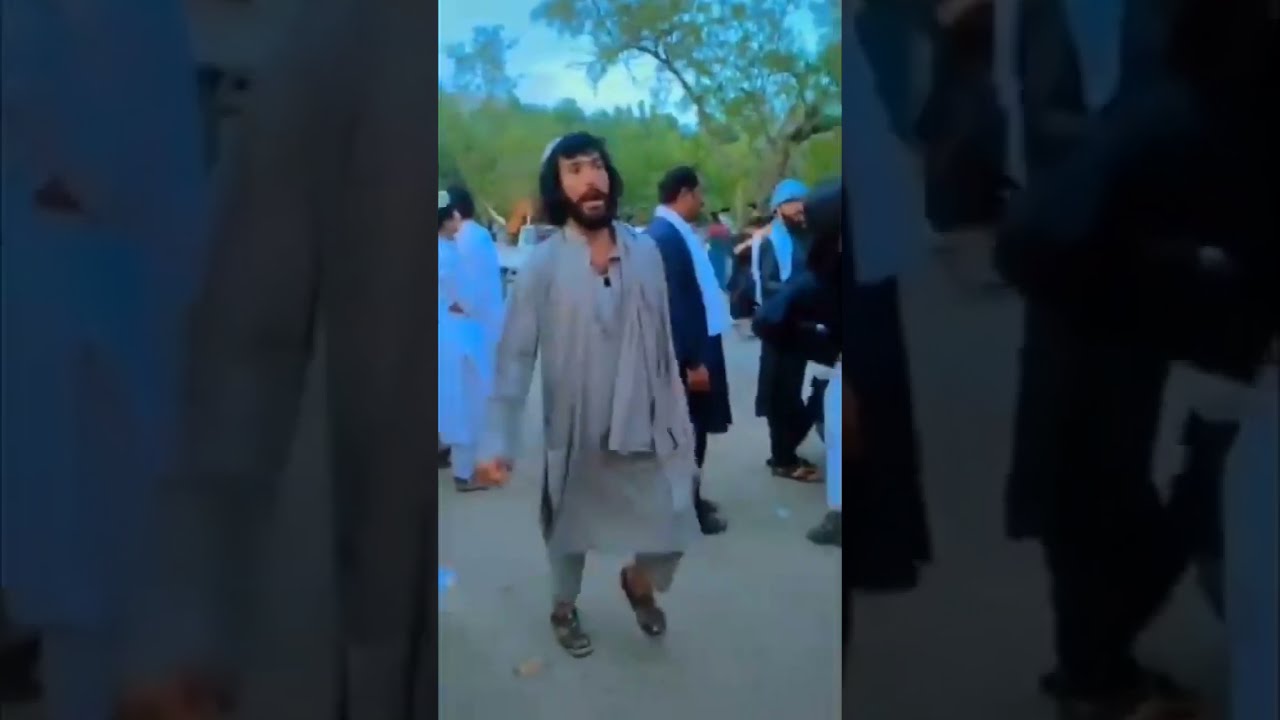The image captures an outdoor gathering of several Jewish individuals, identifiable by their yarmulkes. The central figure is a man with long, dark hair, a beard, and a mustache, dressed in a long gray robe and brown shoes. He stands on a gray surface, possibly a road, in the middle panel of the image—the left and right panels are dark, possibly featuring close-up details from the main scene. Surrounding him are other men, some wearing blue robes and scarves, and others in various types of head coverings like turbans. These men appear to be engaged in a celebratory dance or ritual. The backdrop showcases a bright green forest with several trees, their brown trunks visible, and a partly cloudy, blue sky. The overall mood suggests a religious or cultural celebration.